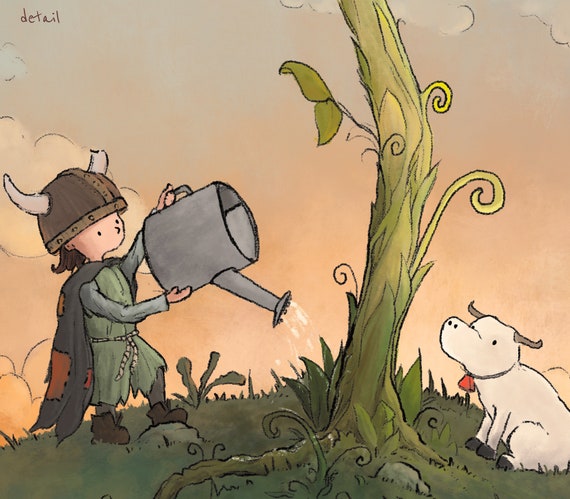In this detailed drawing, a young Viking boy is depicted watering a beanstalk with a large watering can. He is dressed in a tattered green robe with gray long sleeves, tied around the waist with a small rope, and wears a gray cape adorned with tan patches. His Viking helmet sits atop his semi-long hair, and he pairs his outfit with brown boots. The scene includes a small white cow with two horns, little black hooves, and an orange bell around its neck, watching the boy attentively. The background features a slightly pink sky with puffy clouds, suggesting a serene, elevated landscape—potentially a hill. The overall art style and the elements, such as the costume and the beanstalk reaching beyond the picture, add a whimsical and fantastical feel to the illustration.